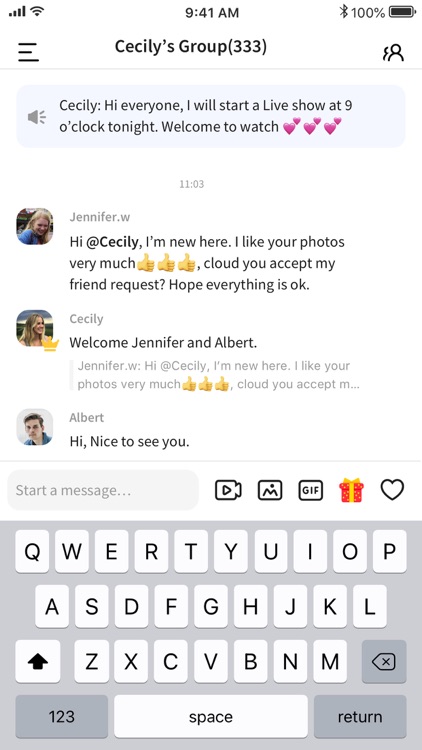The image is a screenshot taken from a mobile phone. It features a white background with primarily black text.

At the very top left corner, there are icons displaying the Wi-Fi signal and cell phone signal strength. At the top center, the time is shown as 9:41 a.m. To the top right, there is the Bluetooth logo, followed by "100%" indicating full battery life.

In the center portion of the screenshot, the text reads "Sicily's Sicily's Sicily's group 333." To the left of this text are three vertical black lines. To the right, there are silhouettes of people.

Below this, the text reads: 
"Sicily hey hi everyone I will start a live show at nine o'clock tonight welcome to watch" followed by heart emojis.

Further down, it shows a timestamp of "1103." Below this, there is a message from "Jennifer W" with an icon of a woman's face, which appears to be that of a Caucasian woman wearing a blue t-shirt. The message says:
"Hi Sicily I I'm new here I like your photos very much thumbs up emojis cloud you accept my friend request hope everything is okay."

Following this, there is a reply from "Sicily":
"Welcome Jennifer."

Next is another message from "Jennifer W" that reads:
"Hi Sicily I'm new here I like your photos very much cloud you accept M…"

Below that, there is a message from "Albert" which reads:
"Hi nice to see you."

Sicily's profile picture shows what seems to be a blonde Caucasian woman staring off to the right, with a home in the background. Albert’s profile picture appears to be a portrait of a white man, focusing on his face.

At the bottom of the screen, there is an input field that says "Start a message…" accompanied by icons for GIFs and images, followed by an on-screen QWERTY keyboard for typing messages.

Overall, the image predominantly showcases black text on a white background, with various user interactions and elements indicating that the screenshot is from a mobile messaging or social media application.